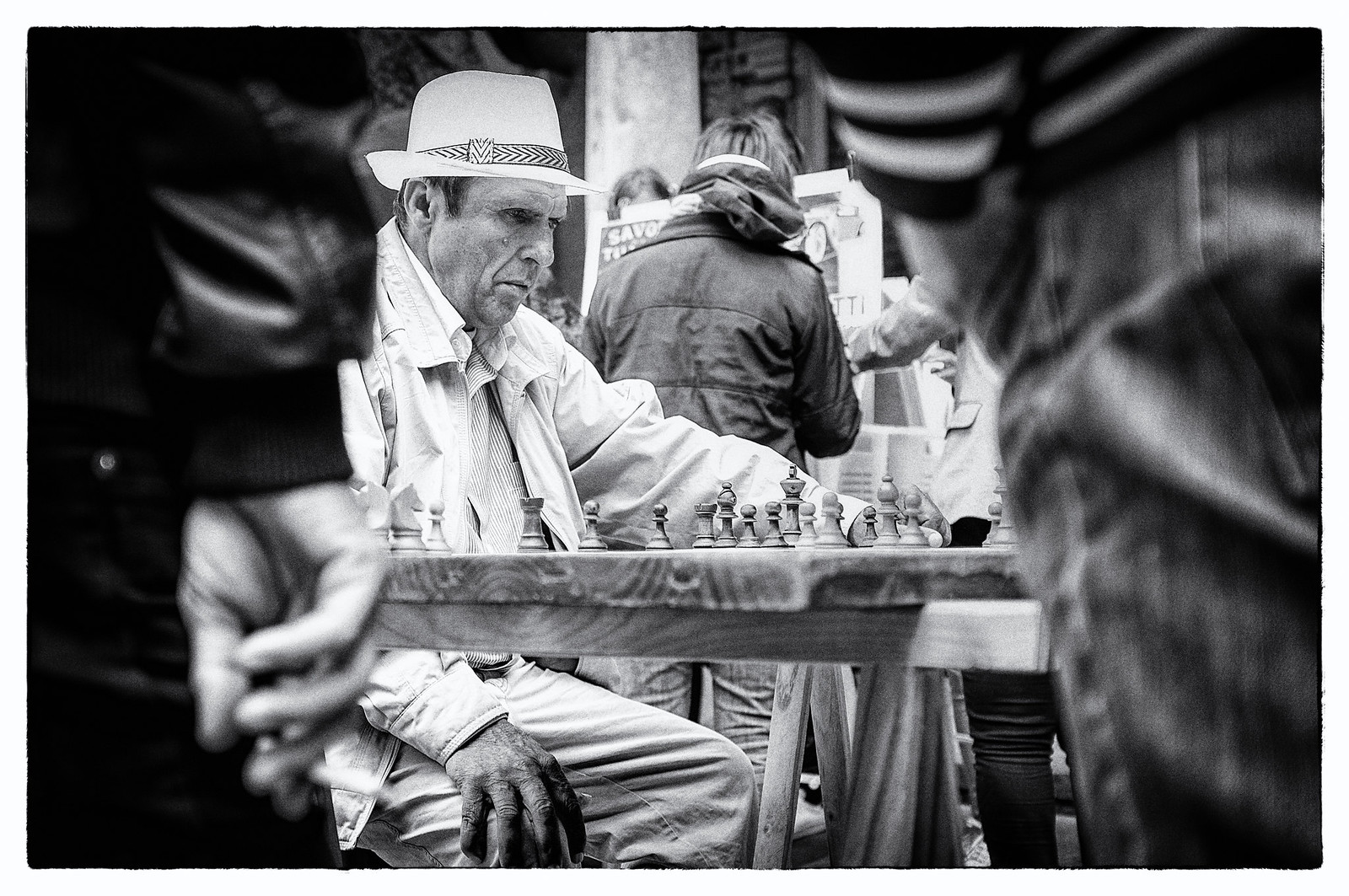This detailed black-and-white photograph captures an older man, likely in a public park, seated at a small, square, wooden chess table. The man, positioned centrally in the image, is deeply focused on a chess game. He is wearing a light-colored outfit, layered with multiple jackets over a shirt, and topped with a hat that has a wide brim, possibly resembling a Cuban-style hat. His attentive gaze is directed at the chessboard, although his opponent is obscured from view by the blurred figures flanking the left and right sides of the frame. These segments depict close-up, blurry portions of other men, primarily showing their hips, arms, and jackets with hands hanging down. In the background, there are a few individuals standing with their backs turned towards the viewer, in front of what appears to be a poster or a piece of artwork. The scene’s monochromatic palette spans black, white, and various shades of gray, contributing to a timeless and contemplative atmosphere.